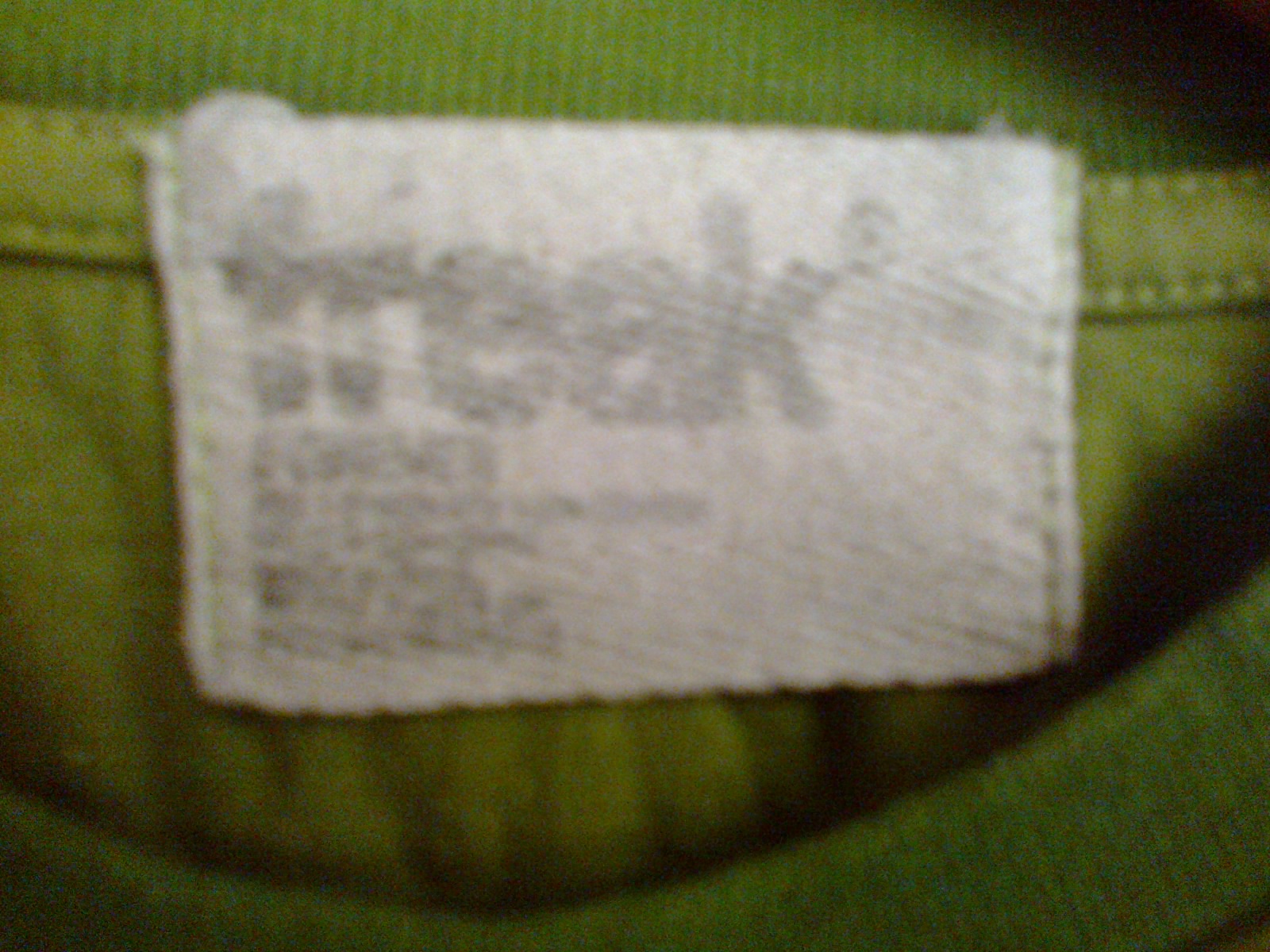A close-up, slightly blurry photo captures a worn clothing label affixed to the neck area of a shirt or sweater. The label, a white albeit dingy horizontal rectangle, prominently displays the word "freak" accompanied by a small copyright symbol. Below this text, faint and indistinct letters suggest the presence of fabric content or size information. The label is securely attached with meticulous sewing machine stitches on both sides and at the bottom. The garment itself is an avocado green, featuring a crew neck neckline that appears folded. At the top of the image, some ribbing from the neckline is visible behind the label.